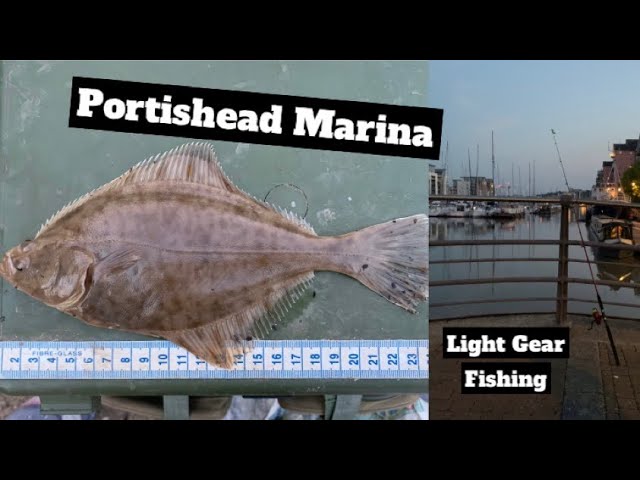The image is composed of two juxtaposed photos with black trim at the top and bottom. On the left is a close-up of a brown, speckled fish with prominent fins along its back, belly, and top. The fish, lying on a green surface, is measured by a tape measure below it, indicating its length of approximately 24 centimeters. A black rectangle with white text above the fish reads "Portishead Marina." On the right side, the scene shifts to a marina, where boats are moored and buildings are visible in the background under a clear blue sky. A fishing pole leans against a railing in the foreground, possibly indicating the vantage point from a boat. Text in a black rectangle at the top reads "Light Gear," with "Fishing" written beneath it in another rectangle.